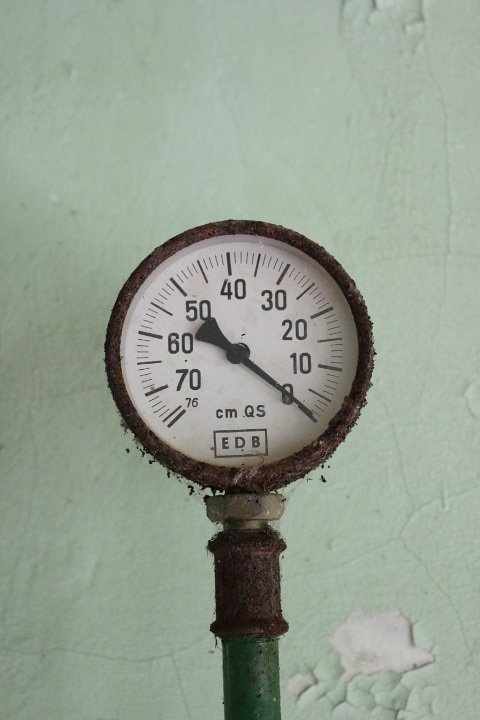This photograph showcases an old-fashioned, weathered gauge situated in front of a green-painted wall. The wall, streaked with age, reveals cracks in the paint, and in the bottom right corner, some chips have exposed the white surface underneath. The focal point of the image is the rusty gauge, which extends from the lower middle to about halfway up the composition. The gauge has a white face bordered by a corroded metal ring. It is marked sequentially from 70 down to 0 in black ink, starting from the bottom left and progressing clockwise. At the bottom of the gauge face, the letters "cmQS" are printed, with "cm" in lowercase and "QS" in uppercase. Below these letters, within a small box, is the abbreviation "EDB."

A thin pointer rests at the zero mark, while the black fanned end of the pointer is positioned between the 50 and 55 marks. The functionality of the gauge remains unclear, leaving its purpose ambiguous—whether it measures pressure, water, or something else entirely is unknown. Beneath the gauge, a screw and additional rusted metal components are visible, leading down to a green metallic pole also marked by flaking and decay. The overall scene evokes a sense of antiquity and neglect, emphasizing the gauge's historical and mysterious presence.